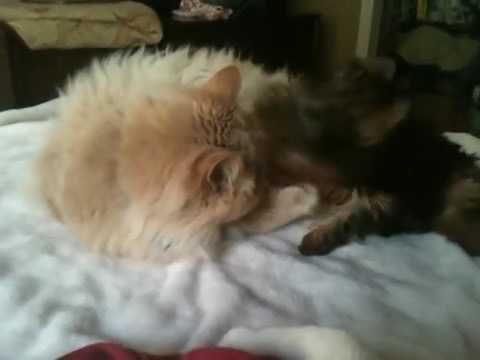The image features two kittens resting closely together on a fluffy, white, rippled blanket that lends a cozy texture to the scene. The kitten on the left has a light whitish-blonde fur with a slightly darker strawberry blonde hue on top of its head, which is pointed toward the camera, ears perked up. This kitten has a soft, long-haired appearance with a paw visible toward the center of the image. Next to it on the right is a second kitten characterized by a darker coat; it has black fur covering its back and legs, with lighter brown tones underneath. This darker kitten appears to be in motion, with its head and one paw slightly blurred, indicating playful activity. The background is indiscernible but seems to include living room furnishings like chairs and tables, rendered indistinct due to the image's blur and poor quality. Both kittens are lying on a red-colored fabric visible at the edge of the blanket, adding a touch of warmth to the scene.